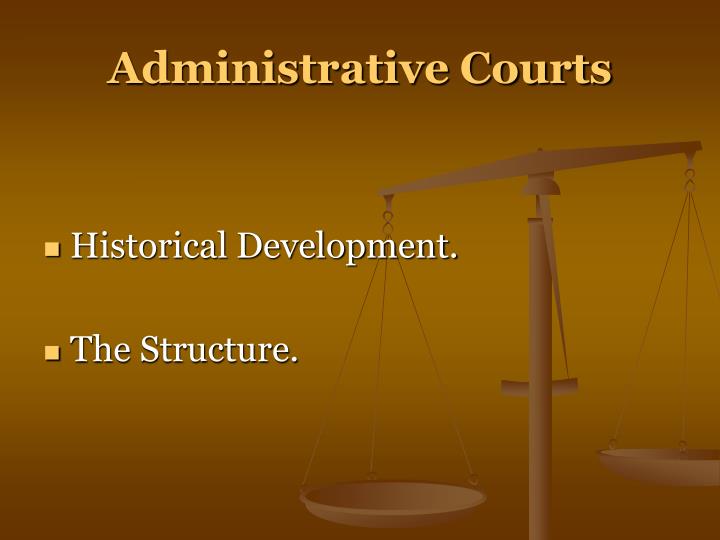The image features a background that transitions from a lighter orange-gold in the center to a darker tannish color at the edges. At the top of the image, in pale beige-orange letters, is the heading "Administrative Courts." Toward the left-middle of the image are two square bullet points in white text: the first reads "Historical Development." and the second reads "The Structure." Each phrase is punctuated with a period. On the right side of the image, towards the bottom right corner, there is a line drawing of the Scales of Justice, with the right plate slightly higher than the left. The overall image combines elements of varying shades of orange, peach, and yellow, giving it an administrative and legal thematic appearance without additional text or imagery.